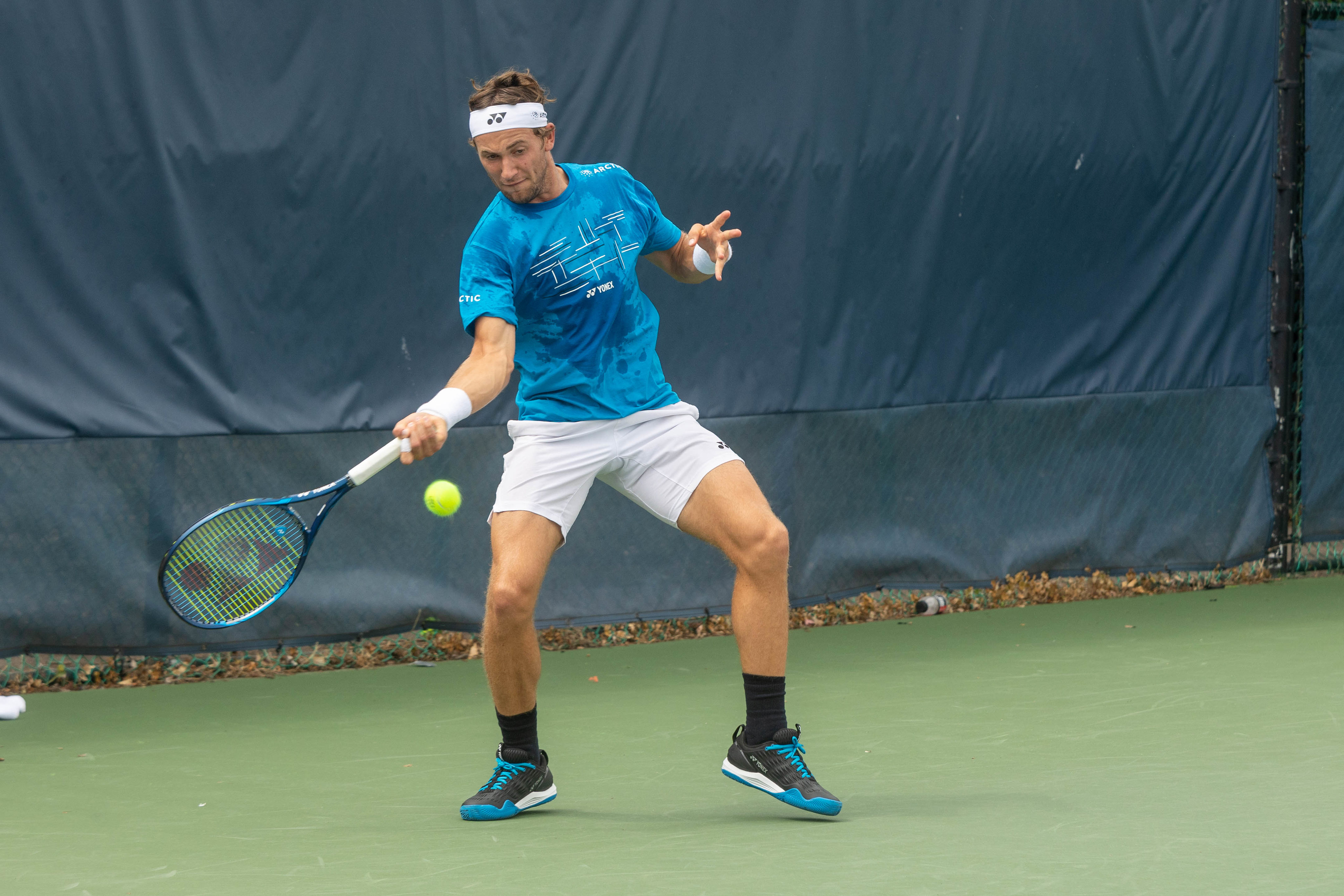The daytime photograph captures a male tennis player on a grass court, poised in a serving position. He is wearing a blue half-sleeve jersey, white shorts, black socks, and blue and black sneakers. His accessories include a white headband on his forehead and white wristbands on both wrists. He has brown hair. The player is holding a tennis racket with a white handle and a yellow net interlaced with a red pattern in his right hand. A yellow tennis ball can be seen in the air near the racket. The background features a blue and black screen that encircles the court, emphasizing the intensity of the match.